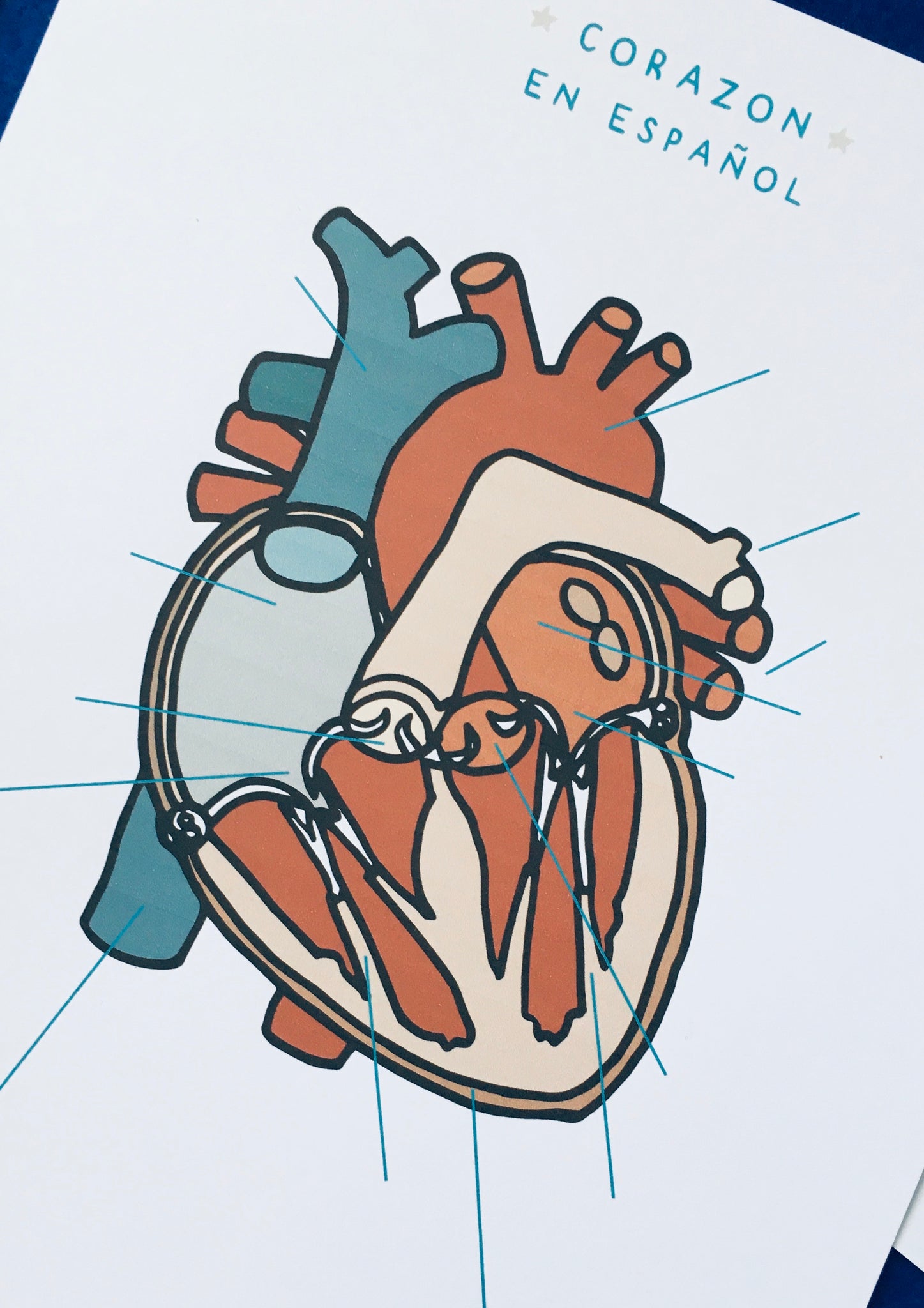The image shows a detailed, cartoon-like diagram of a human heart on white paper, featuring the anatomical shape with visible chambers and ventricles. The heart is illustrated in creams, dark blue, light blue, terracotta, and orangey-brown colors, with blue lines pointing to various sections. At the top of the page, there are two lines of text, "Corazón en Español," flanked by light gray stars at a slight diagonal in the top right corner. The paper appears printed and is set against a blue background, which is visible in the upper corners of the image.